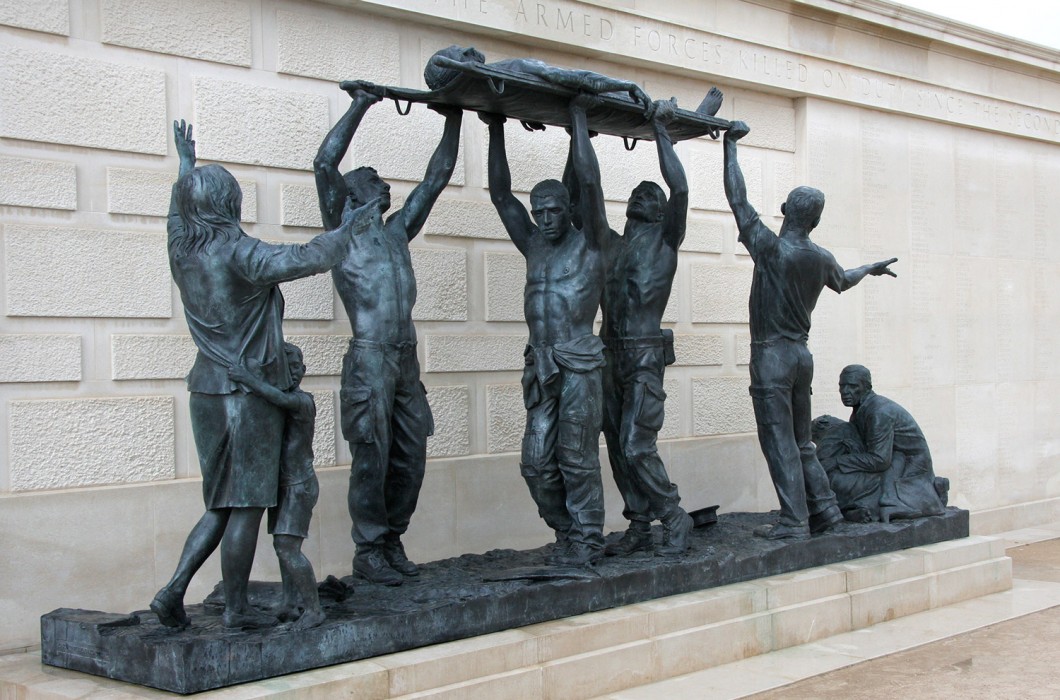This image depicts a detailed and solemn monument set against a backdrop of white stone with brick outlines, possibly located outside a war museum. Central to the image are five statues, intricately carved to represent men lifting a platform or stretcher carrying another figure, likely symbolizing the fallen. Each statue appears deeply serious, contributing to the overall somber mood of the scene, indicative of mourning and respect. 

To the right, another poignant statue shows a man kneeling, tenderly supporting a woman who might represent the mother of a soldier, while nearby, a woman stands with a child hugging her waist, both adding layers of human emotion to the monument. The color palette is muted, with shades of gray, tan, white, and black, enhancing the gravity of the sculpture. The only discernible text, though difficult to read, includes the words "Armed Forces Allied," grounding the statue's dedication to military personnel. The entire sculpture appears meticulously designed to capture the collective grief and honor associated with the fallen soldiers.